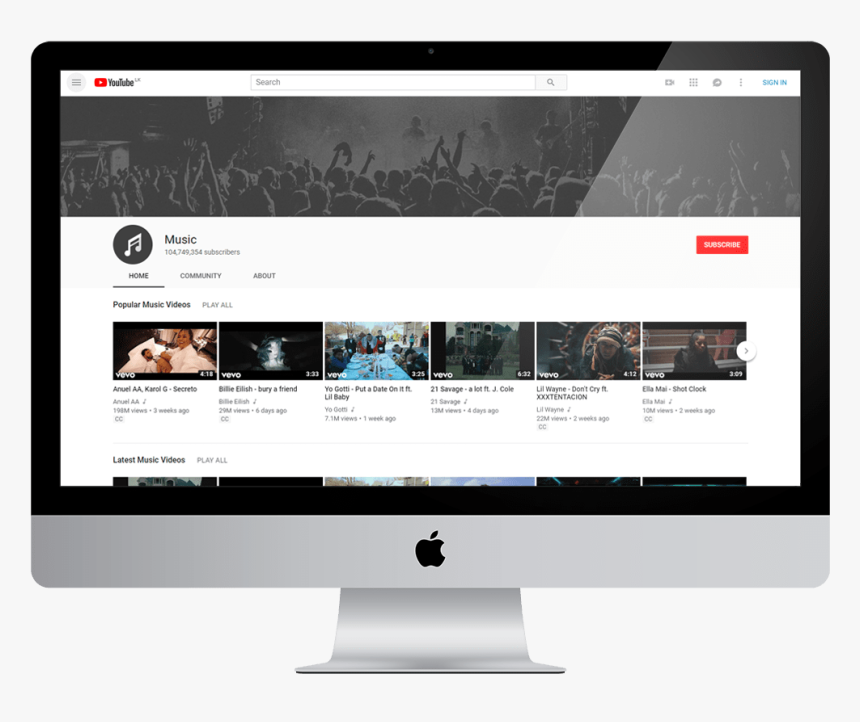In this image, a desktop Mac computer is prominently displayed, showcasing the YouTube Music platform on its screen. The interface indicates that YouTube Music has an impressive 404,749,354 subscribers. The screen also features navigational tabs including Home, Community, About, Popular Music Videos, Latest Music Videos, and a Play All button. Additionally, the iconic Apple logo is clearly visible on the Mac desktop, emphasizing the brand's presence. The overall setup reflects a modern and tech-savvy environment.